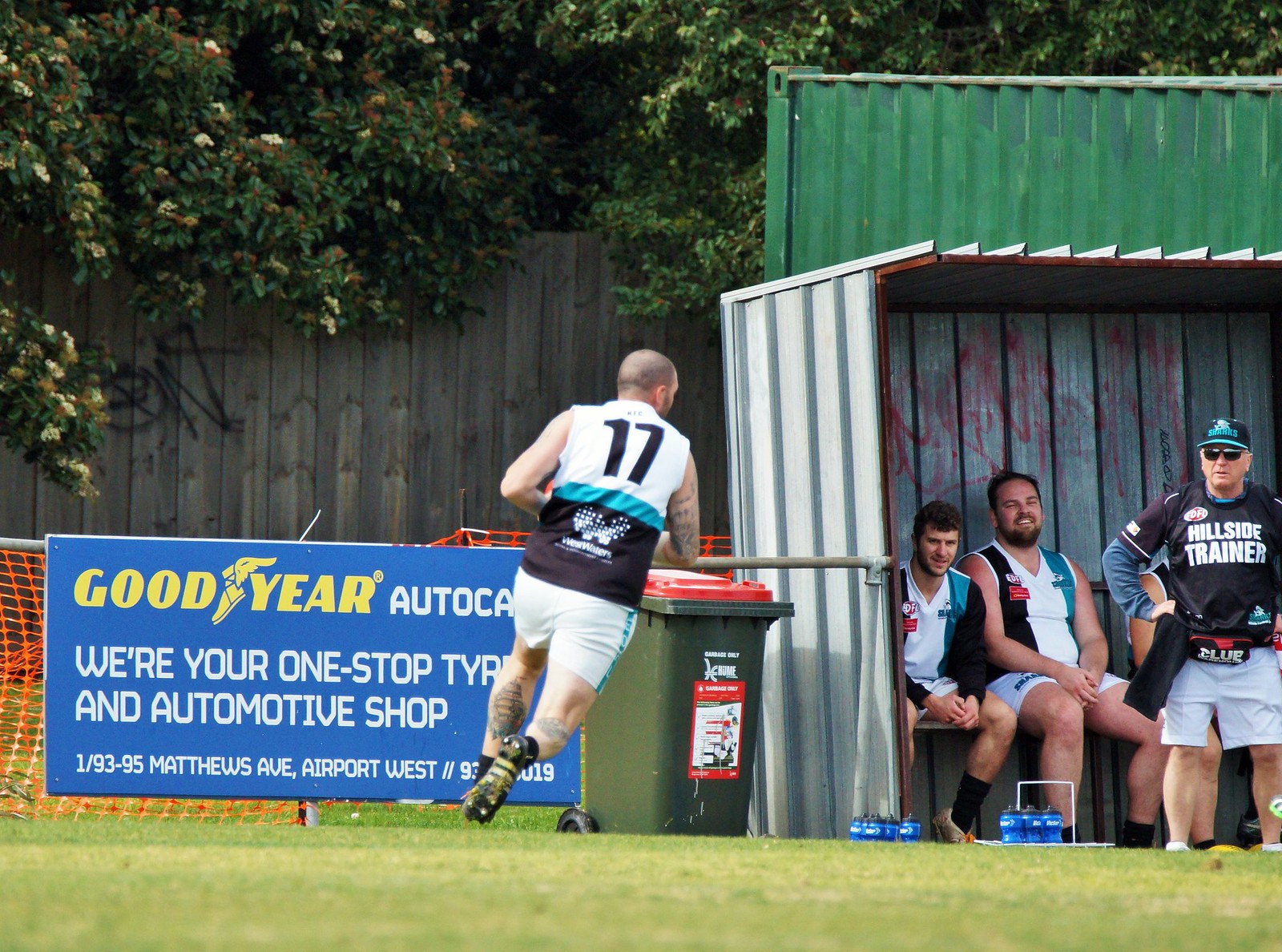The image captures a person running on a soccer field towards a steel dugout. The runner, seen from behind, wears a white and blue striped jersey with the black number 17 and white shorts. To the right, in the dugout, are five men, three of whom wear matching uniforms. Another man, labeled as the 'Hillside Trainer,' is in shorts, a hat, and glasses, standing near two containers of blue water bottles. A green trash can with an orange lid and a blue signboard reading "Goodyear Auto Care, where your one-stop tire and automotive shop, 1/93 to 95 Matthews Ave, Airport West" are attached to a metal pipe railing. In the background, a white plank fence, partially obscured by tree branches and leaves, displays black graffiti. Additionally, an orange net fence, hooked to the metal railing, separates this setup. The scene is set on a partly cloudy day, with the men in the dugout appearing to be engaged and relaxed, smiling at the running player.